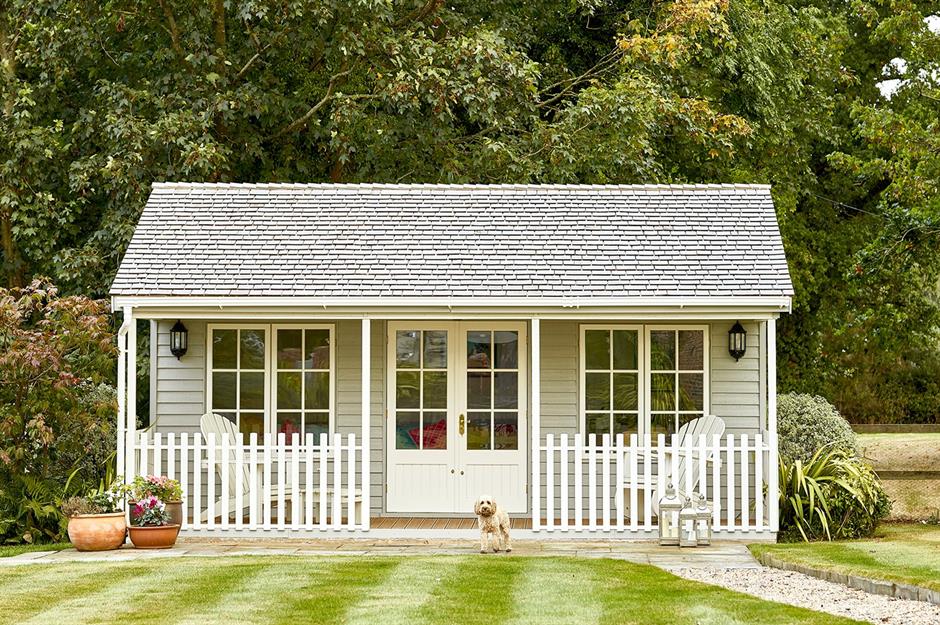The image depicts a small, modern one-story house, centrally positioned with almost equal spacing on all sides. The house features a white front door with windows, flanked by two sets of double windows also framed in white. A white picket fence borders the property, and a neat walkway lined with white stone gardening rocks leads to the house. On the front porch, there are two white chairs. 

In front of the house, posing beside the fence, is a small white poodle staring directly at the camera. The landscape is meticulously maintained, with manicured green grass and several terracotta plant holders. The background is dominated by large trees with lush green leaves, creating a serene and secluded atmosphere. Notably, there appears to be a reflective surface suggesting a possible body of water towards the lower right corner of the image.